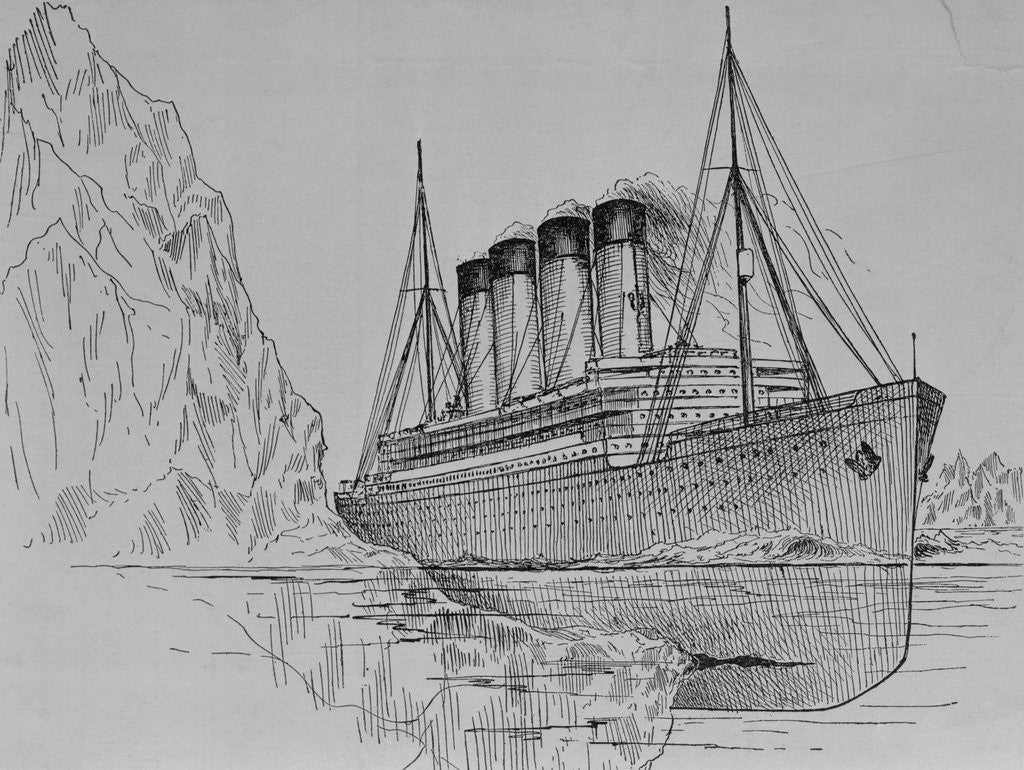This is a detailed black and white line drawing rendered with crosshatching, depicting a distressed ship reminiscent of the Titanic. The drawing captures a striking scene both above and below the waterline. 

At the ship's center, four large smokestacks are illustrated in great detail, with etched shading to highlight their three-dimensional form. The smokestacks culminate in large black cylindrical tops, releasing varying amounts of smoke: minimal from the first smokestack to the rear, with the largest plume emanating from the last smokestack at the bow. The ship itself is intricately lined with windows, rows of balconies, and feature two prominent masts, one at the fore and one at the aft. 

Beneath the surface, we observe a significant gash in the hull where the ship collides with a glacier, depicted by small square windows extending down the hull. The left side shows a massive glacier cutting into the hull, inflicted by an unseen underwater segment of the iceberg—a dangerous obstacle for the ship. The drawing contrasts stark white icebergs, possibly implying an icy landscape, against the gray-toned paper background, enhancing the drama of the scene. Altogether, this highly detailed illustration vividly captures the tragic fate of the ship in a monochrome palette.